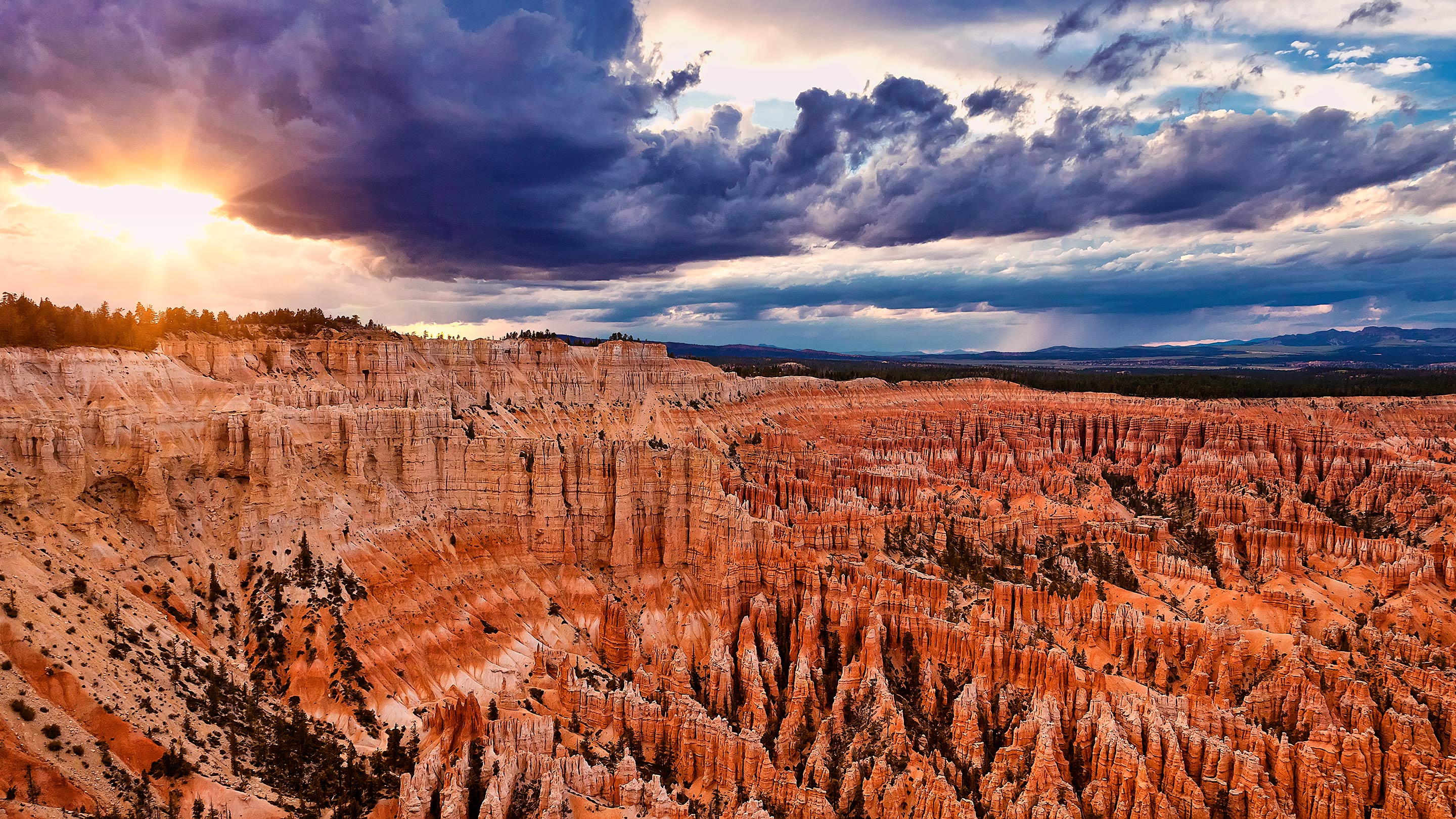The image captures an expansive, vibrant canyon scene reminiscent of the Grand Canyon, possibly Cedar Breaks or Bryce Canyon. The rocky cliffs display striking layers of orange, red, and white sediment, creating a visually arresting geological feature. The photograph, taken from an aerial perspective, provides a clear and detailed view of the terrain, showcasing striated rock formations with individual lines visible in the sediment. Throughout the canyon, dark spots suggest the presence of sparse vegetation, with some trees notably growing on the left side of the image and in the distance.

The sky, covering the upper portion of the photo, is a dramatic tapestry of blue, purple, and dark clouds, hinting at recent rainfall. The setting sun, positioned on the left, peers out from behind the clouds, casting its rays across the landscape and creating shadowy forms within the clouds. Puffy clouds, ranging from white to dark gray, populate the sky, allowing glimpses of the blue sky to shine through, particularly in the center and the right. The entire scene is bathed in a warm, reddish-orange hue, likely enhanced in post-editing, adding to the photo's vivid and picturesque quality.